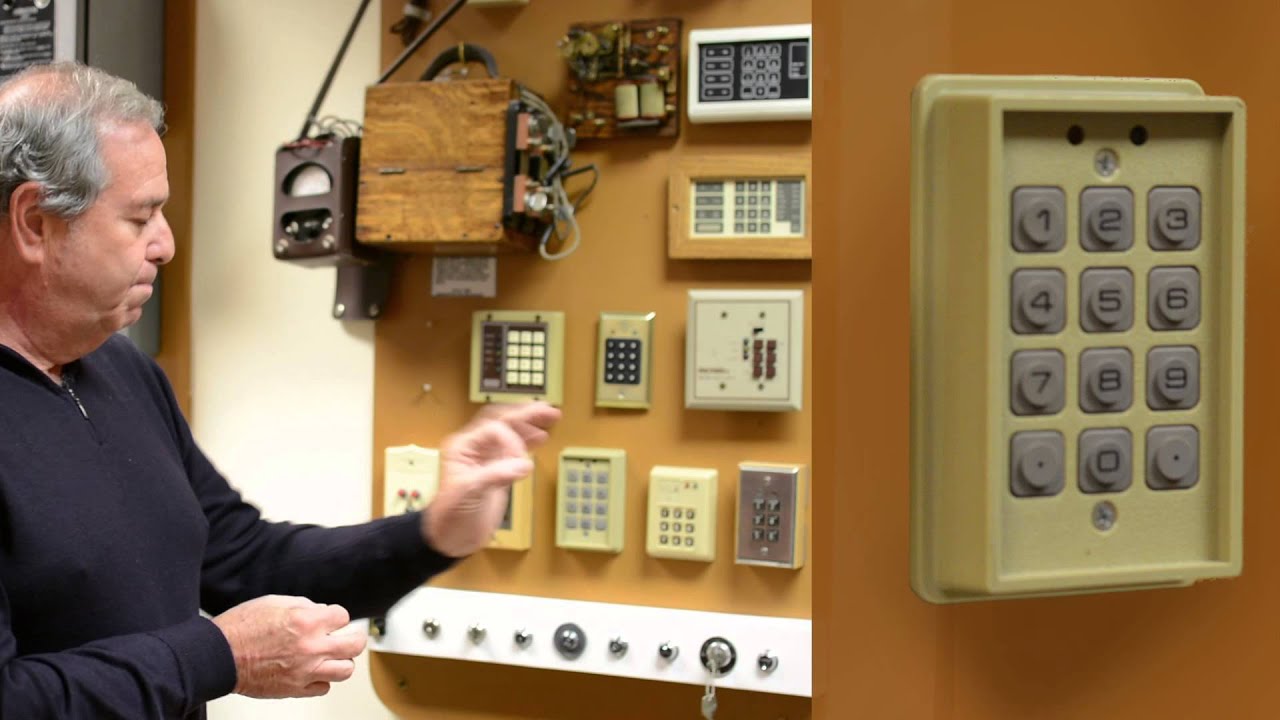In this combined landscape-oriented image, we see two color photographs side-by-side. The left photograph features an older white man with gray hair, a bald spot, and a black sweater. He’s standing in front of a board displaying approximately ten different garage or security keypads in various sizes, colors, and widths. The keypads are neatly arranged, with approximately eight on the bottom two rows and two additional units on the upper right. Above the left side of the board, there's a wooden box structure with multiple plug-ins. The man, with eyes partially closed and a grimace on his face, appears to be pointing at some of the devices.

The right photograph, in portrait orientation, is a close-up of one of these keypads. This particular keypad is beige with numbered buttons in gray, arranged in four rows from 1 to 0. Each number is encircled and set against a square background, with the entire keypad outlined in yellow. The style of both images leans towards photographic representationalism realism, capturing the details with precision and clarity.